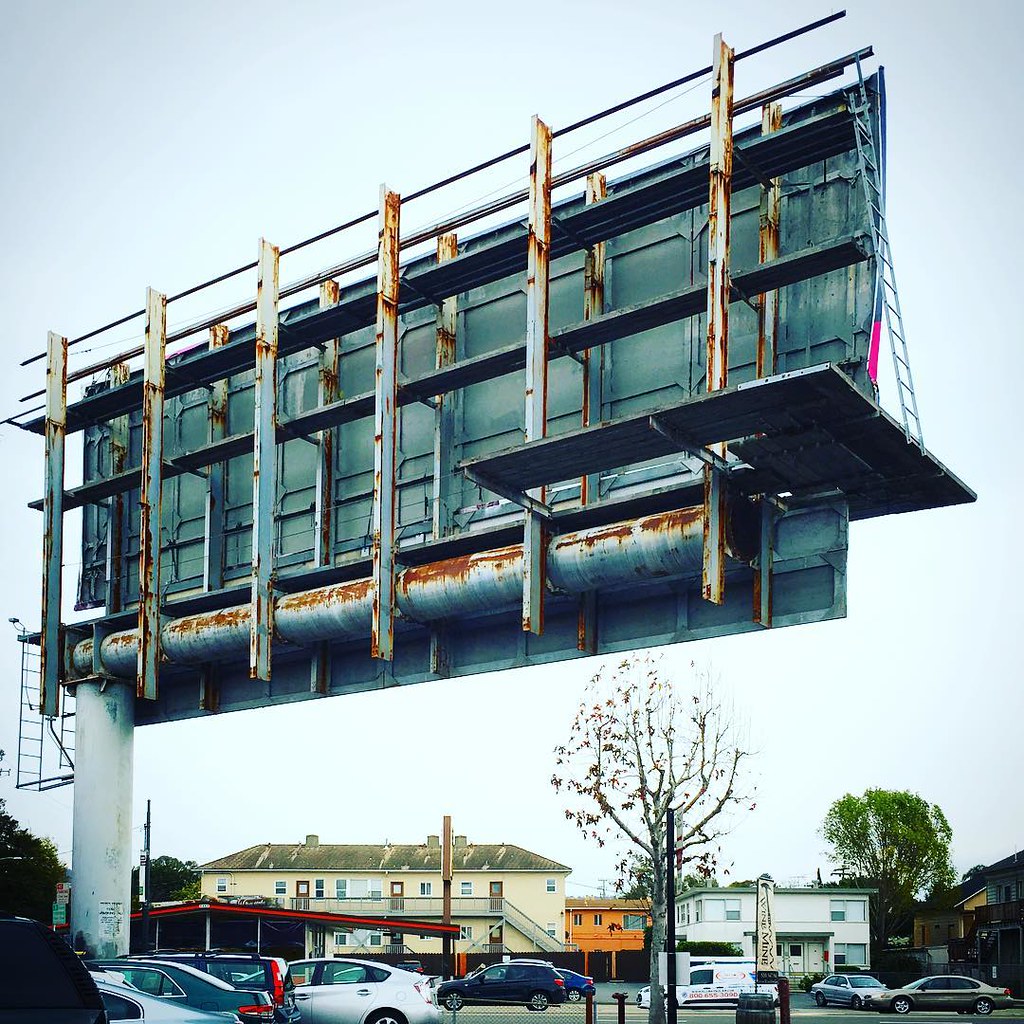A detailed street view featuring the skeletal back of a rusted billboard, showcasing its rusty vertical and horizontal struts. The billboard is devoid of any advertisements, revealing a platform and a ladder attached to its weathered support tube. Below, there's a residential building with an accompanying parking lot filled with several cars. To the side, two contrasting trees are visible: one lush and green and the other barren, signaling the onset of fall for the latter.